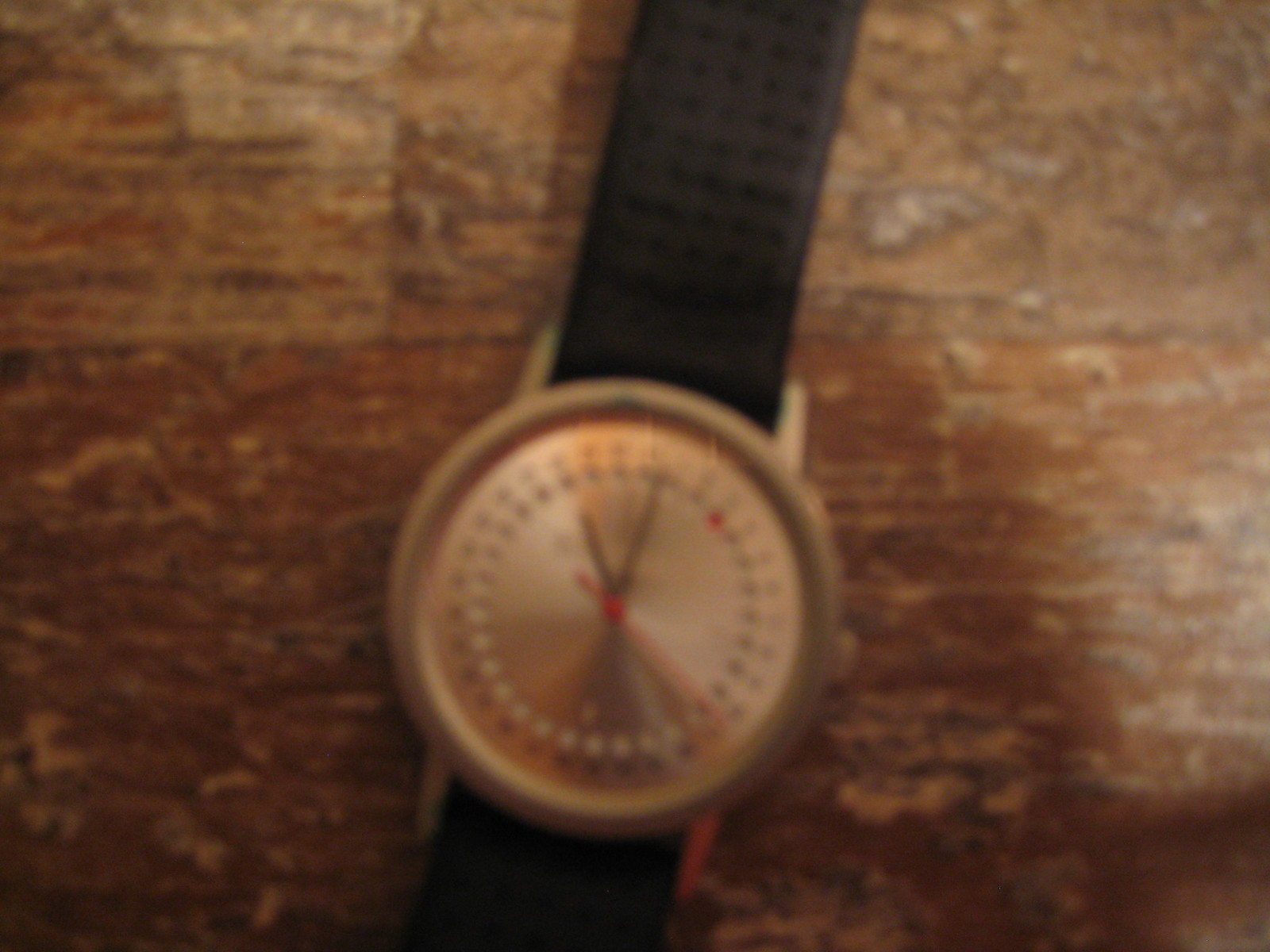This photograph, although of low quality due to its significant blurriness, depicts a wristwatch. The watch features a black band and a gold casing. It has three hands—the hour and minute hands indistinctly positioned, suggesting the time could be 11:00, 4:30, or 6:30—and a red second hand. The watch rests on a distressed, old-looking wooden table, adding a rustic touch to the scene. Despite the lack of clarity, the contrast between the sleek watch and the aged table is evident.